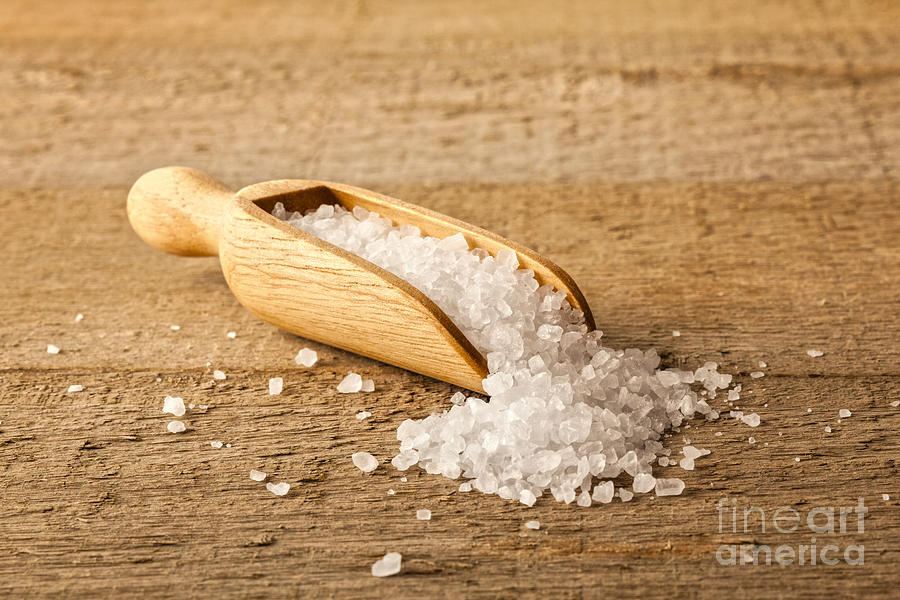The image features a detailed close-up of a light brown, smoothly carved wooden scoop filled with large chunks of white salt. The scoop is positioned prominently at the center of the image, resting on an unfinished, medium tan-colored wooden table with a slightly rough texture. The salt, which appears to be crystalline and coarse, spills generously from the scoop onto the wooden surface, creating a vivid contrast between the white salt and the brown hues of the wood. The text "Fine Art America" is subtly present in the lower right-hand corner, indicating that the image may be a professionally taken photograph, possibly intended for an art website or magazine.